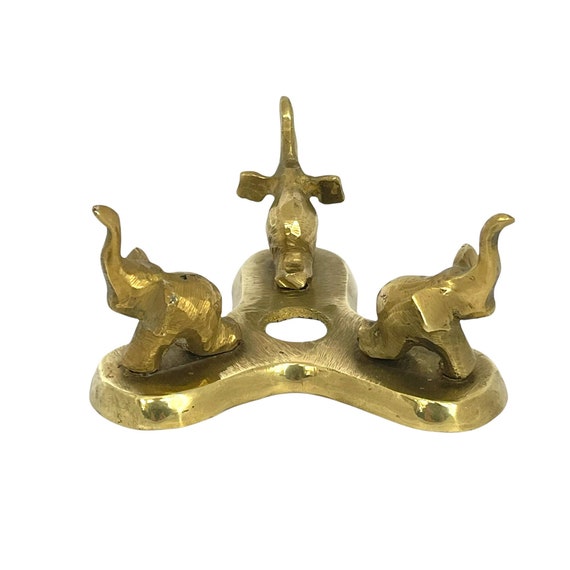The image features a brass statue against a plain white background, sculpted into a Y-shaped structure, somewhat resembling a fidget spinner or a pie chart. The statue consists of three chiseled golden or brass elephants, each with their trunk raised and lacking detailed features. These elephants are welded onto each of the Y's arms. The base of the statue also shares this brass build, and the center of the Y-shape has a circular opening, revealing the white background behind it. Notably, the elephants exhibit signs of wear, with black and brown discolorations on various parts of their bodies, adding a touch of character and history to the piece.